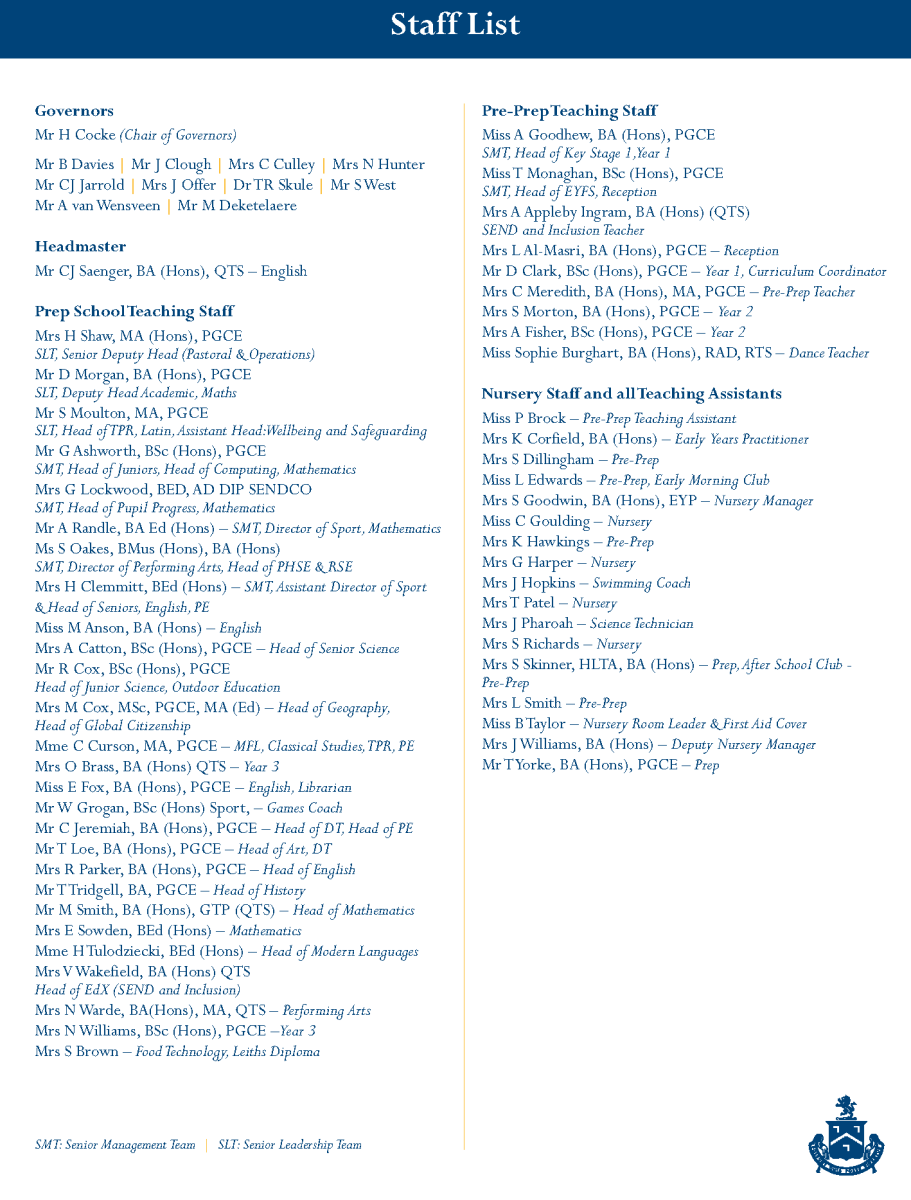The image displays a detailed staff list for a prep school, prominently labeled "Staff List" in white text within a large navy blue box at the top. The list begins with a section titled "Governors," featuring five individuals: Cook, Davies, Jarrod, Van Wensreen, and one unnamed person. Following this is the designation "Headmaster," indicating the school's leader.

Beneath, the list transitions to a section labeled "Prep School Teaching Staff," signifying a comprehensive roster of educators for the preparatory students. A solitary listing labeled "CMT" appears below this staff roster, standing alone without a specific category.

Divided by a vertical line running down the center, the right side of the image details the "Pre-Prep Teaching Staff," followed by a segment for "Nursery Staff and All Teaching Assistants," indicating educational personnel for younger, nursery-aged students. 

The entire staff list is written in blue text on a white background and includes ample white spaces for clarity. The footer of the image features an emblematic crest, styled in navy blue, which resembles those typically found on school uniforms, further emphasizing the prestigious nature of the institution. The crest includes an illustration of a house with additional elements beneath it, reinforcing the elite and traditional image of the prep school.